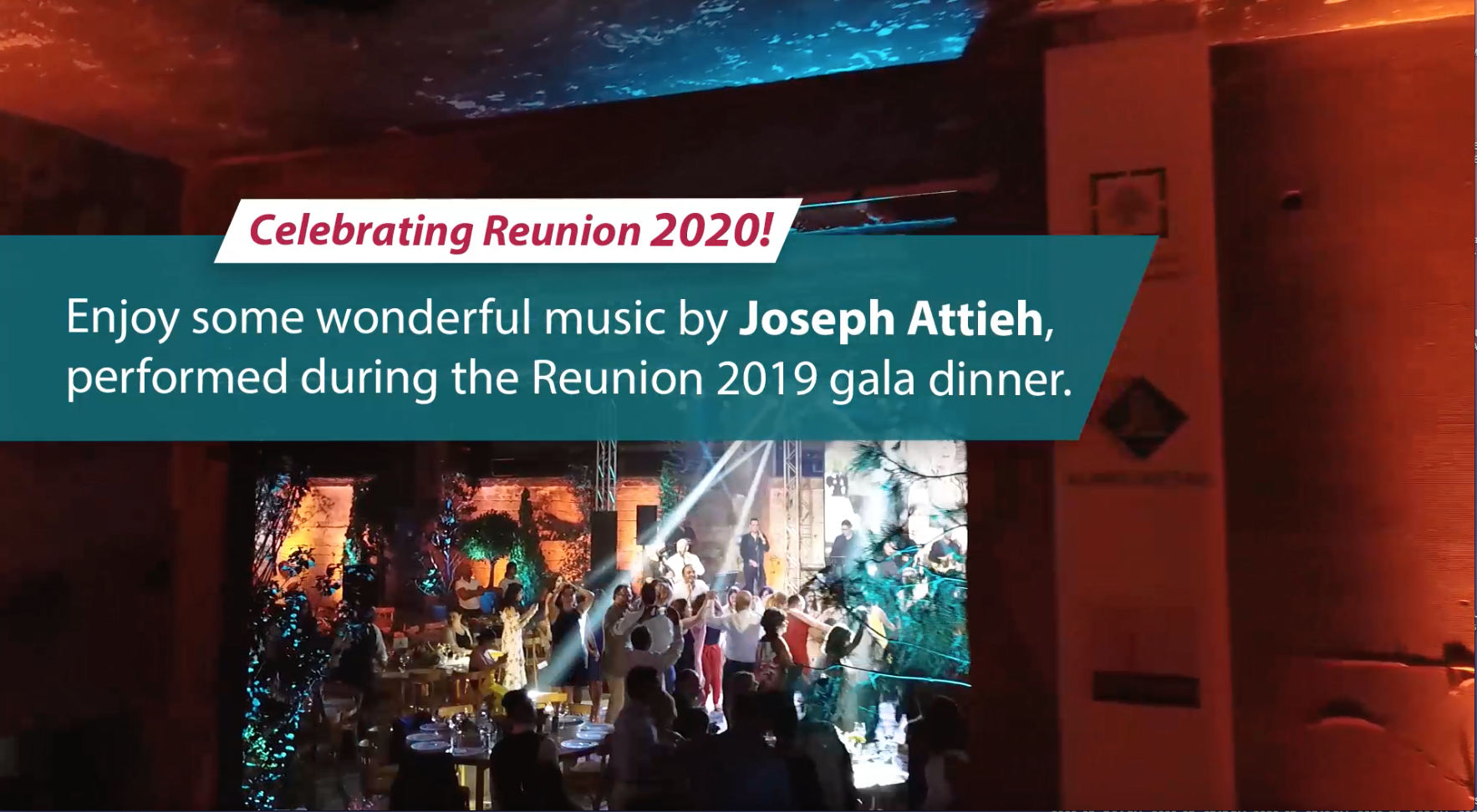The image captures a lively and colorful scene from a celebratory event titled "Celebrating Reunion 2020!" The title is prominently displayed in red text on a light beige rectangular banner. Below this, in a similarly styled narrow rectangle that stretches from the middle left to the center of the image, are the words in white text: "Enjoy some wonderful music by Joseph Attieh performed during the Reunion 2019 gala dinner."

The background features a blue and red tinted ceiling and reddish-looking walls, an effect created by ambient lighting. The scene showcases a lively restaurant or club setting with a stage area where performances occur. Tables with seated guests surround a busy dance floor filled with people enjoying the music. The image appears to have a digital or painted aesthetic that contributes to its vibrant, mood-lit atmosphere. Splashes of oranges, greens, and other vivid hues add to the festive and energetic ambiance, making the overall picture colorful despite the dim lighting.